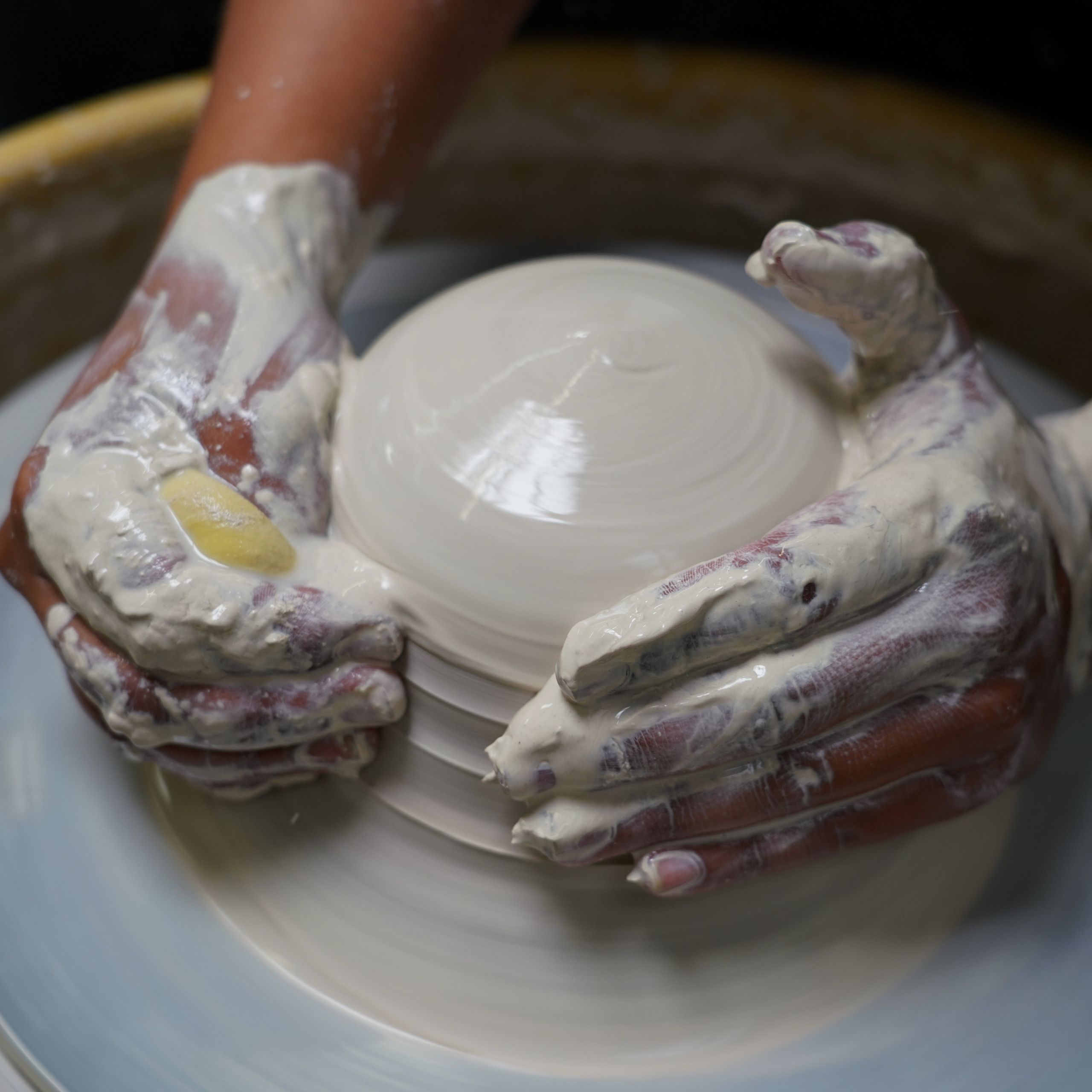The image captures a person with tan or possibly dark skin molding pottery on a spinning wheel. Their hands, partially coated in wet clay, skillfully shape a creamy white or pale yellow ceramic piece that appears to be in progress, possibly cylindrical in form. The right hand holds a yellow sponge, aiding in the sculpting process. The pottery wheel, which shows a motion blur indicating its rotation, is light blue with a yellow outer rim. The background is entirely black, providing a stark contrast that highlights the pottery activity focused in the center. Only parts of the forearm and hands are visible, immersed in the delicate art of pottery-making.